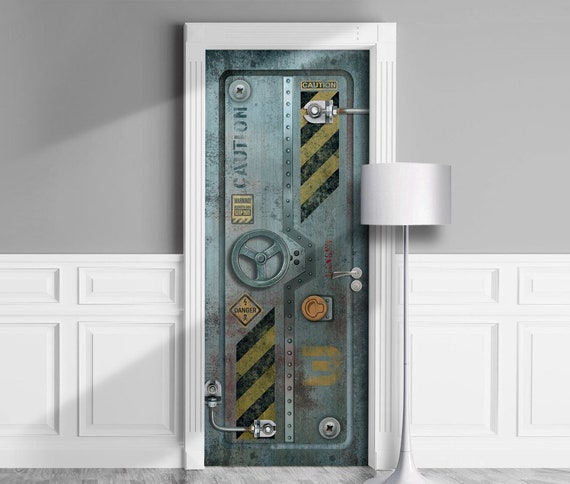The image showcases a digitally created scene reminiscent of a computer game environment. The setting features a distinctive door, resembling a vault or submarine hatch, complete with a circular turn wheel handle for unlocking and locking. This metal door is light green, adorned with various caution signs, including a vertical "Caution" stencil in the upper left corner, black and yellow hazard stripes, and another sign near the wheel warning of electrical danger. The door also features numerous metal reinforcement rivets, bars, and screws, enhancing its technical appearance.

Surrounding the door, the wall is divided into an upper gray portion and a lower white section, which is designed to look like decorative wood paneling, mimicking the appearance of cabinets. A tall, thin lamp with a white lampshade stands to the right of the door, extending about two-thirds up its height. The lampshade, though not actively illuminating the scene, suggests that an additional light source from the upper right of the image contributes to the overall lighting.